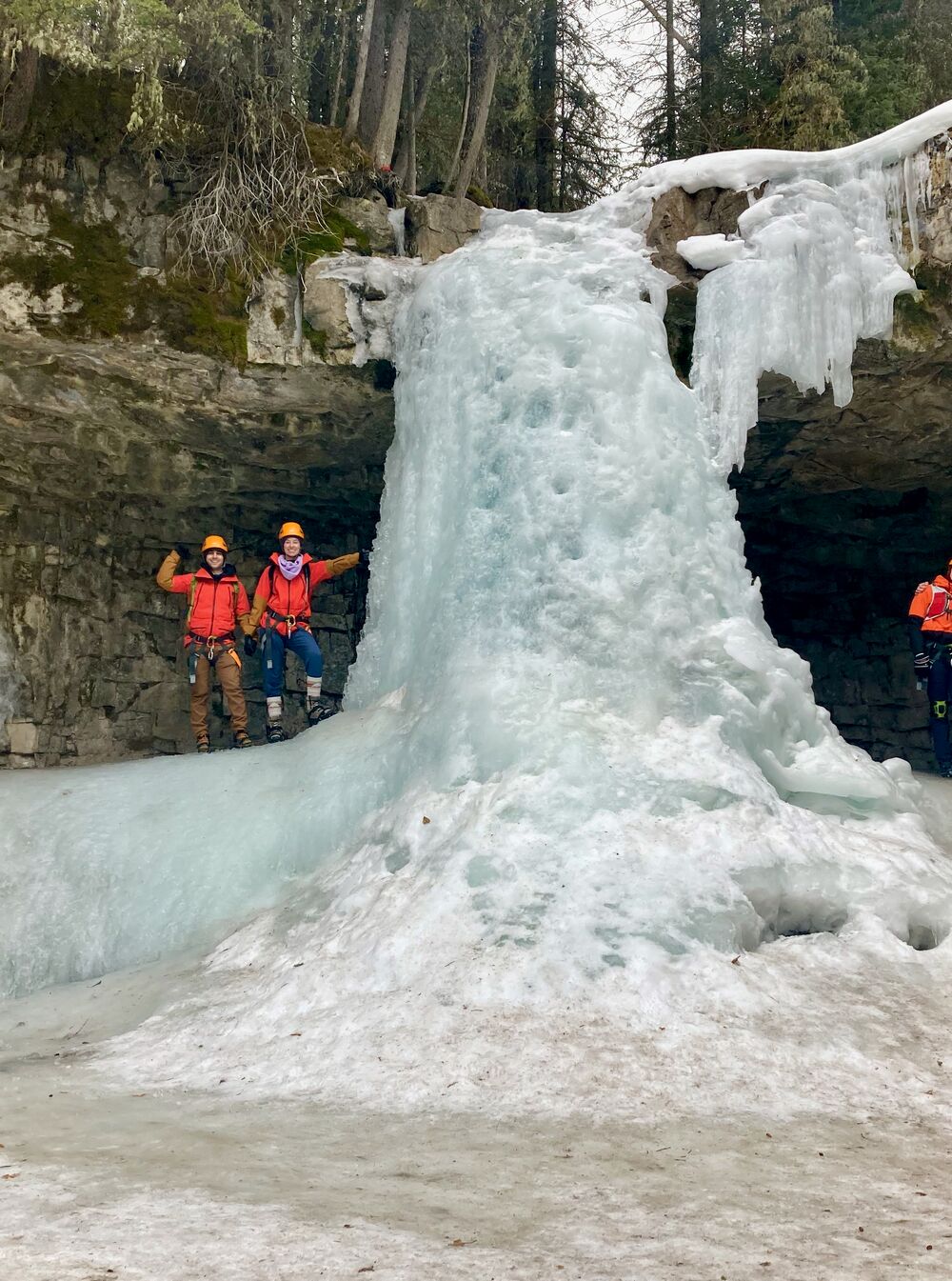This captivating photograph features a frozen waterfall emerging from a forest backdrop. The waterfall, now an immobile cascade of ice, appears to have been halted mid-flow, descending from the moss-covered rocks above into a stony alcove. The ice exhibits various shades of white, with subtle hints of blue, gray, and even lilac, interspersed with brown speckling scattered throughout.

In the foreground, three hikers in neon orange jackets and yellow hard hats add a burst of color against the icy landscape. On the left side of the waterfall, a smiling man, dressed in brown pants, waves at the camera while the woman beside him, wearing a lavender scarf and blue jeans, gently touches the frozen cascade. On the right edge of the image, another person in an orange jacket and black pants stands partially out of frame, their face turned away from the camera.

Above the frozen spectacle, trees still holding onto their leaves frame the scene, suggesting the forest is not completely dormant despite the winter freeze. The intricate details of roots emerging from some trees and the green algae on the boulders add to the rich, natural tapestry captured in this remarkable moment.